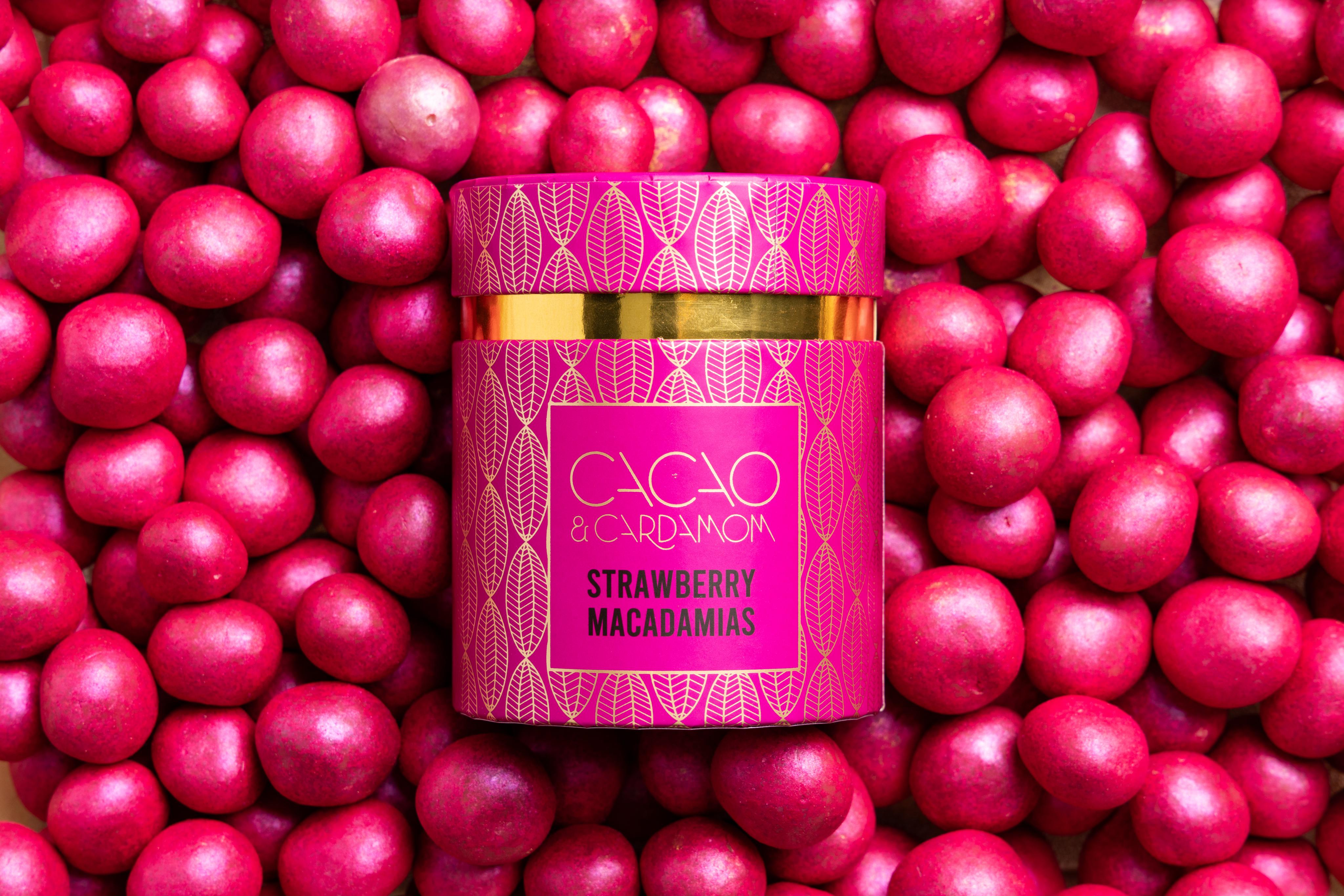The image features a visually striking arrangement of glossy, pink-coated macadamia nuts, suggesting a gourmet snack labeled as "Strawberry Macadamias." These shiny macadamias fill the entire background, creating a vibrant and textured backdrop. In the center of this display lies a pink cylindrical container detailed with repetitive up-and-down leaf patterns and accented by a gold band encircling its middle. The canister boasts gold lettering that reads "Cacao and Cardamom Strawberry Macadamias," hinting at the luxurious flavor combination within. The bright and reflective nature of the composition enhances the allure of the product, making the macadamias gleam under the light.